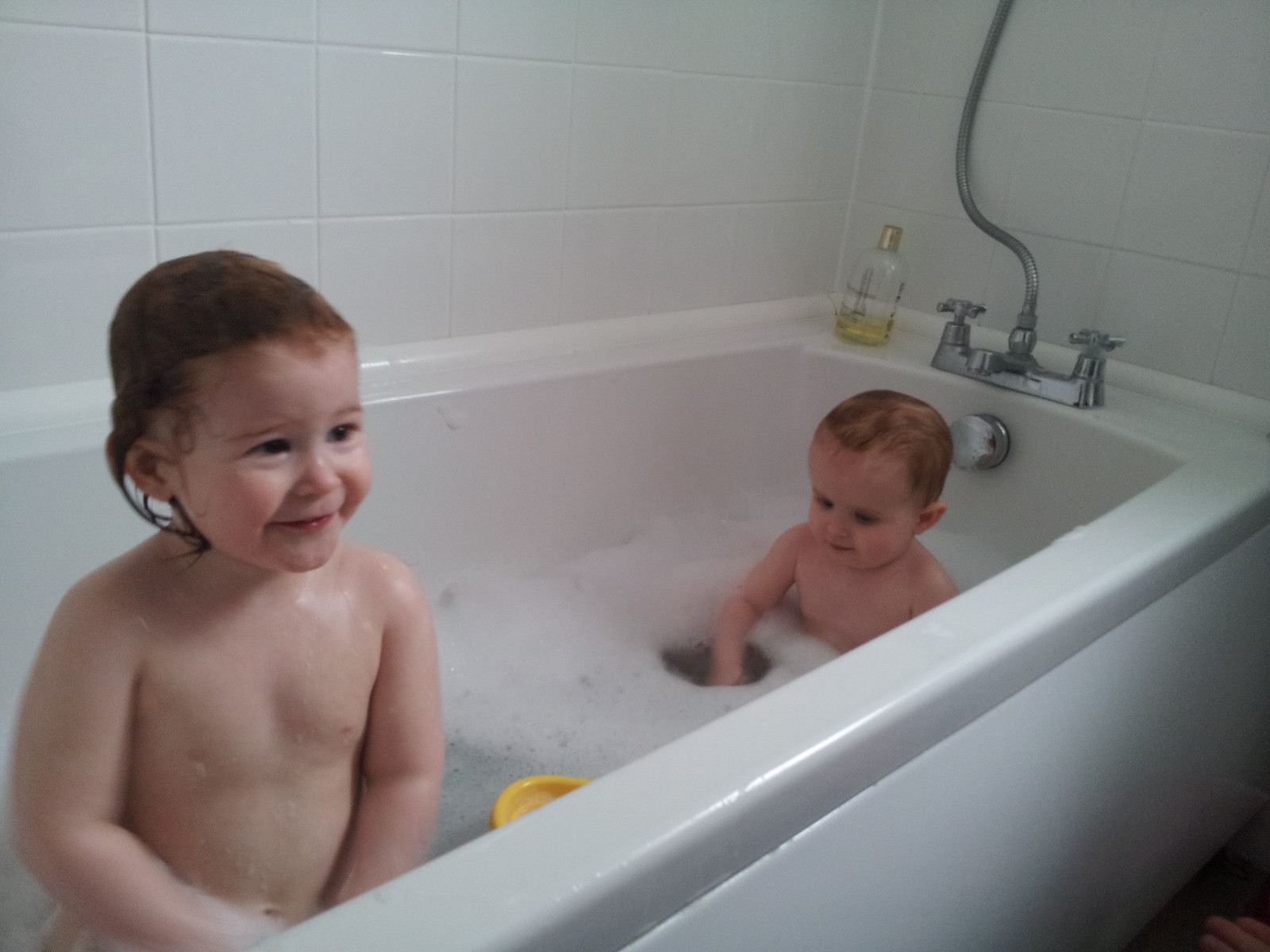The image depicts two children enjoying a bubble bath in a white porcelain bathtub with white tiled walls. The bathroom fixtures, including the spigot and handles, are silver. In the foreground, the older child, who has slicked-back, light brown (almost reddish) hair, looks out of the tub and smiles towards someone off-camera. This child appears to be wet and is positioned on the left side of the tub from the camera's perspective. Floating in the water near them is a yellow toy. Further down the tub, nearer to the spigot, sits a younger child, likely a toddler, with short light brown hair. This smaller child is engrossed in the bubbles, smiling and playing with their hands submerged in the froth. On the edge of the tub behind the children is a mostly empty clear bottle with black writing and a silver cap, containing what appears to be a yellow liquid. The overall scene is filled with bubbles, splashes of playful joy, and the clean, bright aesthetic of the bathroom enhances the lively and cheerful atmosphere.